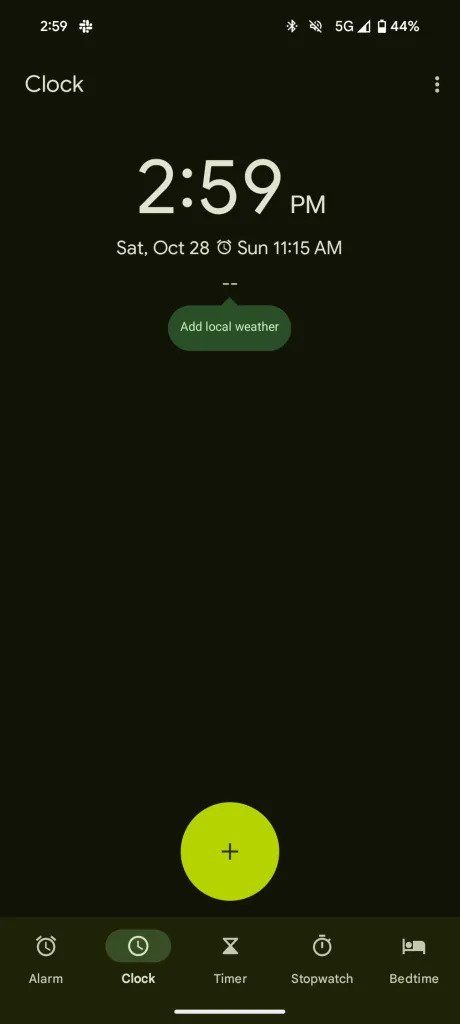The image depicts a detailed black interface screen with various elements and icons. 

In the top-left corner, the screen shows a battery indicator at 44%, a signal strength icon marked "5G," and a clock displaying "2:59 PM," followed by the current day and date "Saturday, Oct 28." Next to the clock, there's an alarm clock symbol indicating an upcoming alarm set for "Sunday, 11:15 AM." In the top-right corner, there are three vertical dots suggesting a menu or additional options.

Below, in the center of the screen, there's a space prompting the user to "Add local weather" with the text in white, while a green oval, followed by two dashes, appears next to this text.

At the bottom portion of the screen, there's a yellow circle with a grey plus icon inside it, placed against a dark gray background with a tint of green. Further down, different functional icons are lined up, each accompanied by descriptive text in white. These include "Alarm" with an alarm clock icon, "Clock" with a clock icon, "Timer" depicted as a sand capsule, "Stopwatch" shown with a stopwatch icon, and "Bedtime" indicated by a bed icon. At the very bottom middle of the screen, there's a white bar crossing the entire width.

This thorough description captures the intricate details and color schemes present in the image interface.